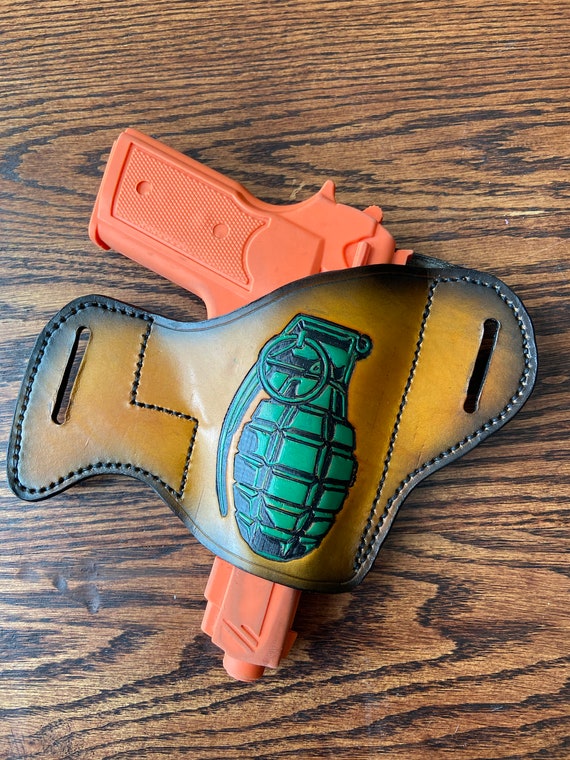The image showcases a bright orange toy gun, resembling a water pistol, seated in a leather-like holster on a wooden surface. The wood is light brown with a dark brown grain pattern, adding a rustic texture to the scene. The holster, designed with burnished edges that transition to black, is yellow-brown and features visible stitching on both sides as well as belt slits without a belt. In the center of the holster, a bright green grenade is carved into the material, creating a stark contrast against the orange gun. The gun, which is slightly worn with a brownish nozzle area, is positioned downward and a bit to the left, adding a dynamic angle to the composition.